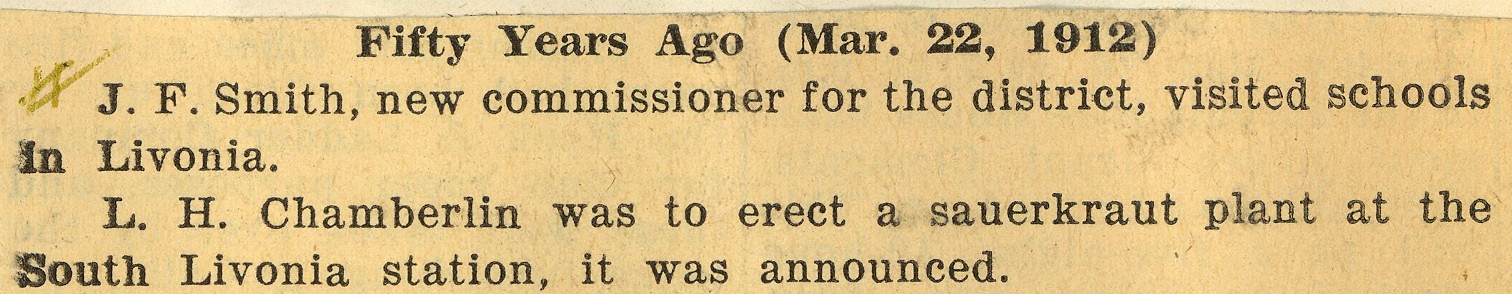The image depicts a vintage newspaper clipping from the 1960s, preserved in a narrow, horizontal orientation. The aged paper has a dark beige, almost dingy brownish appearance, characteristic of its timeworn state. The black text remains legible and reads, "50 years ago, March 22, 1912," signifying that the clipping likely dates back to 1962. The article details two historical notes: "J.F. Smith, new commissioner for the district, visited schools in Livonia," and "L.H. Chamberlain was to erect a sauerkraut plant at the South Livonia Station, it was announced." The clipping shows signs of its journey through time, featuring a smudged section of text and a peculiar, possibly accidental brownish pen mark to the left of J.F. Smith's name, adding to its vintage charm.